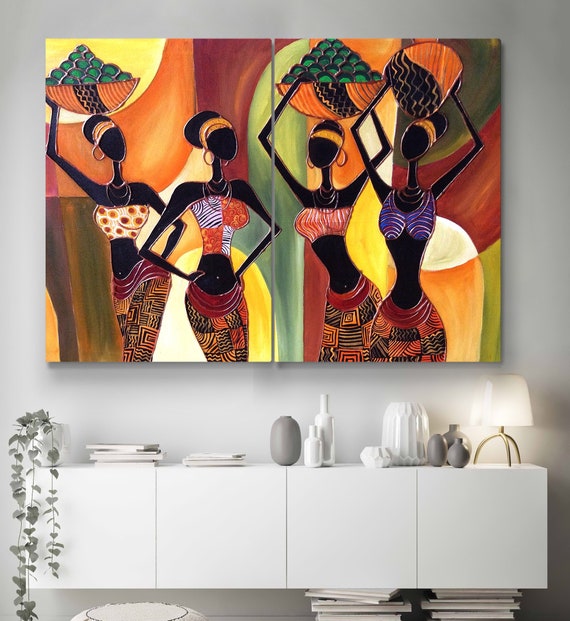The image showcases an intricately decorated interior of a room with a focus on a white, floating cabinet in the lower third, supported by stacks of books at the bottom right. The cabinet has four sections and is adorned with a variety of objects, including a white potted plant with trailing vines, two stacks of books, a smooth jar, two bottles, another white jar, and three pottery-like items. On its far right edge stands a white, shaded lamp. Above the cabinet hangs an eye-catching two-paneled wall art against a white wall, vividly colored in orange, yellow, and green. The artwork portrays four African women adorned in colorful bandeau tops and skirts, with three carrying fruit bowls on their heads and one holding an unidentified object. The women also wear headbands and hoop earrings, adding to the vibrant and dynamic feel of the painting. The overall interior exudes a balanced blend of minimalist color tones and striking visual art, creating an engaging and harmonious decorative setting.